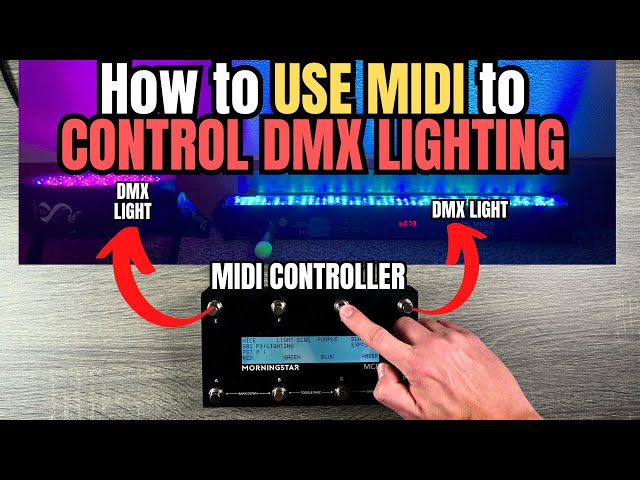The image features a detailed guide titled "How to Use MIDI to Control DMX Lighting" with a predominantly white, yellow, and red text banner at the top. Below this header, a sleek black MIDI controller, resembling the size of a cell phone, is positioned on a gray wooden surface. The controller is labeled "MIDI Controller" in white text and displays a screen with a light blue background and black writing, showing the brand "Morningstar." The device has several silver buttons across its top and bottom, with a person's hand interacting with the third button from the left via their forefinger, while the thumb rests on the side of the controller. Two red arrows emerge from the top corners of the device, each pointing upward to the text "DMX light." In the background, the image includes additional graphics: a round container filled with purple material on the left and a rectangular board with neon green lights and a knob on the right.